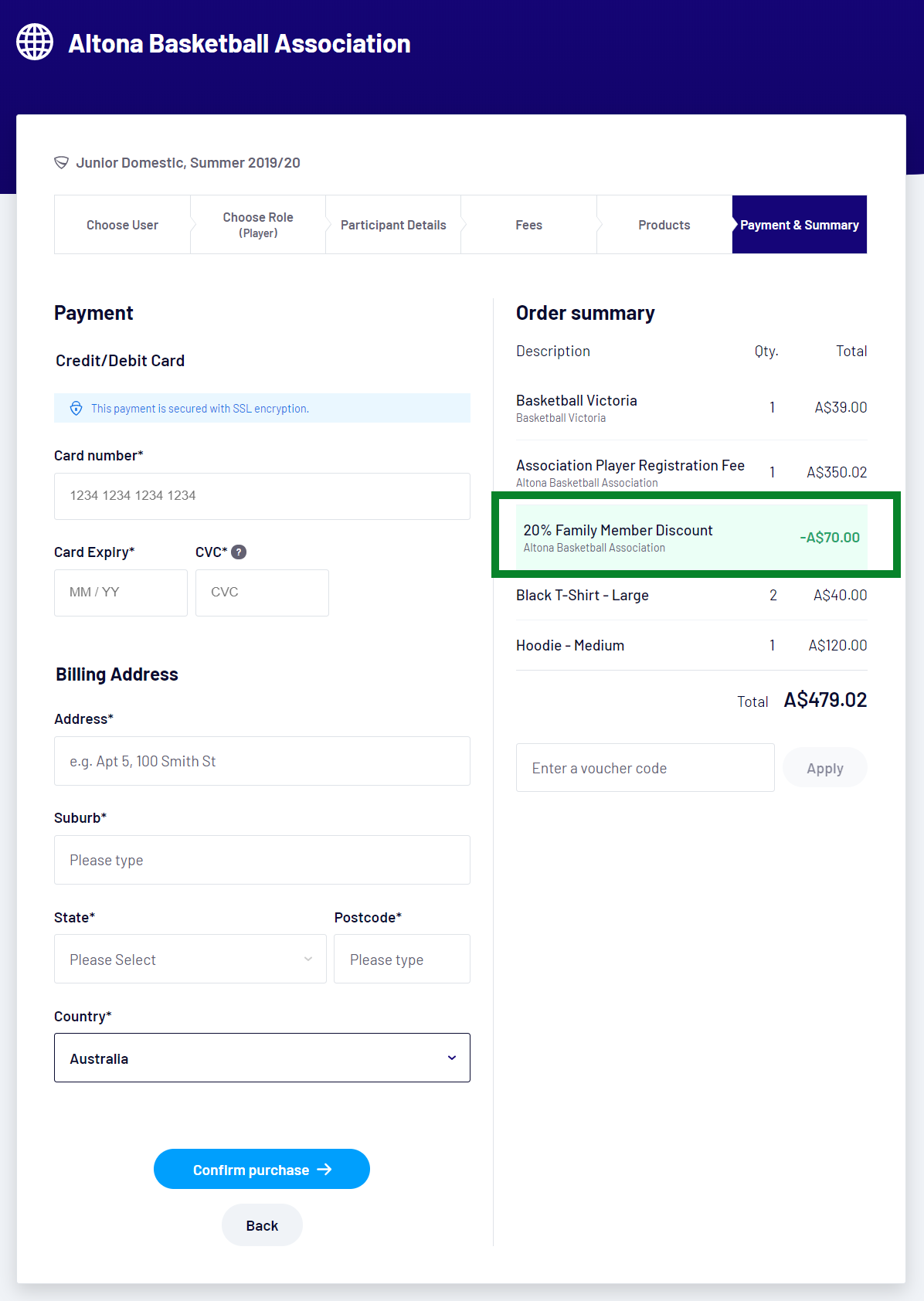This image is a screenshot from an online registration and payment page for the Altona Basketball Association's Junior Domestic Summer 2019/20 season. The webpage allows users to choose their role and details, as well as input participant information, fees, and products, before proceeding to payment.

The payment section includes fields for credit or debit card information, billing address, and country selection, displaying "Australia" by default. Users need to confirm their purchase by clicking the corresponding button, and a back button is also present for navigation.

On the right side of the page, there is an order summary. The summary includes:
- **Basketball Victoria (Quantity: 1)**: $39.00
- **Association Player Registration Fee**: $350.02
- **20% Family Member Discount**: -$70.00, highlighted in a green rectangle.
- **Black T-Shirt Large (2)**: $40.00 ($20.00 each)
- **Hoodie Medium**: $120.00

The total amount due amounts to $479.02.